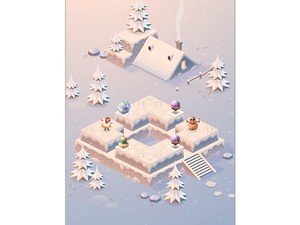The image is a digital print or graphic showcasing a surreal winter scene. Central to the artwork is the upper part of a house, mostly buried under deep snow, with only the roof, chimney, and top window visible. The house is surrounded by a landscape dominated by snow and ice, with a distinct pattern of square or diamond-shaped objects arranged below it. Some squares feature small human figures standing on them, reminiscent of video game characters. White trees, layered in three sections to form a tapered point, are scattered throughout the scene, adding to the wintery ambiance. The color palette is primarily white, with shades of light blue and light purple, enhancing the frosty atmosphere. This striking image blends elements of a snow-covered house, pixelated structures, and tiny characters, creating a unique and whimsical winter wonderland.